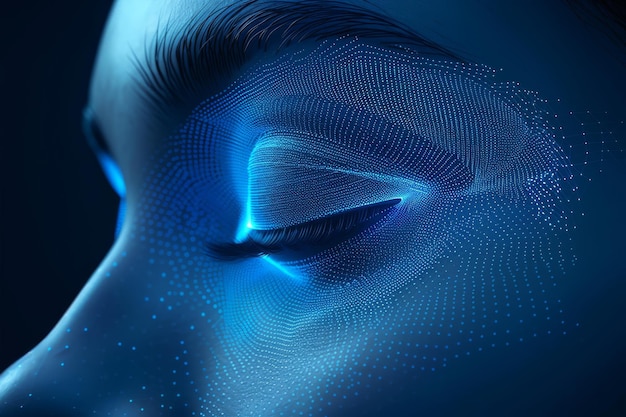This rectangular, computer-generated image, wider than it is tall, portrays a close-up profile of a woman's face, captured from above her eyebrows to just below her nose. The face is facing left against a uniform black background, enhancing the striking luminescent effect. Her eyes are closed, fringed with long black eyelashes, and her eyebrows are also distinctly dark. The face is adorned with an array of uniform white or light blue luminescent dots, giving it an almost manufactured appearance. These dots are particularly concentrated around the eyelids, creating a bright, glowing effect around the eyes and the edges of the nose, which also appears notably luminescent. The overall color palette leans heavily towards blue, contrasting sharply with the black background, and contributing to the image's iridescent quality, which may suggest it is an artistic rendering or heavily edited photograph.